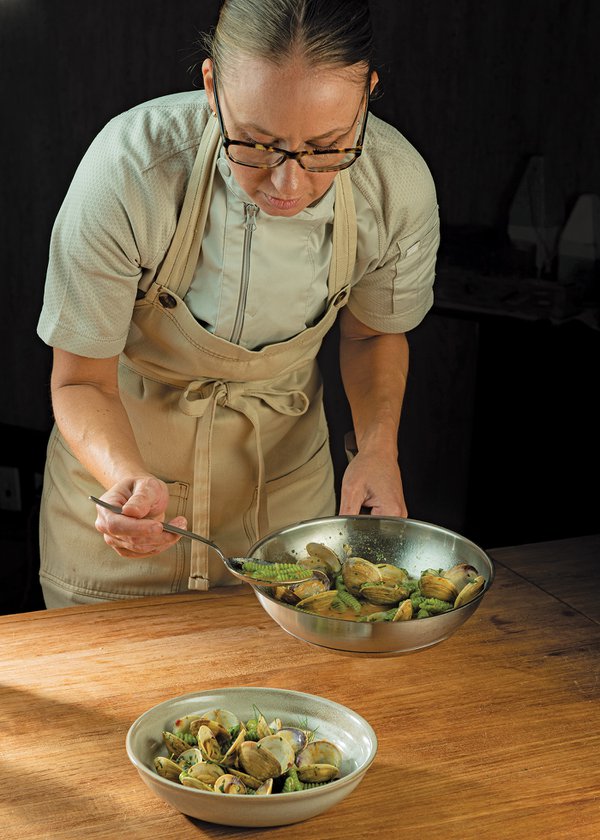This photograph features a woman who appears to be a chef focused intently on her culinary task. She has short black hair that is tied back and wears dark-framed glasses. Her attire includes a white, zippered shirt beneath a beige apron. She is leaning over a wooden, brown table, holding a silver pan in her left hand and a spoon in her right. The pan contains a dish of opened and cooked clams mixed with some green vegetables. She is in the process of spooning this mixture into a half-filled, shiny beige clay bowl that is sitting on the table in front of her. Her concentration on the task suggests a meticulous effort in plating the dish.